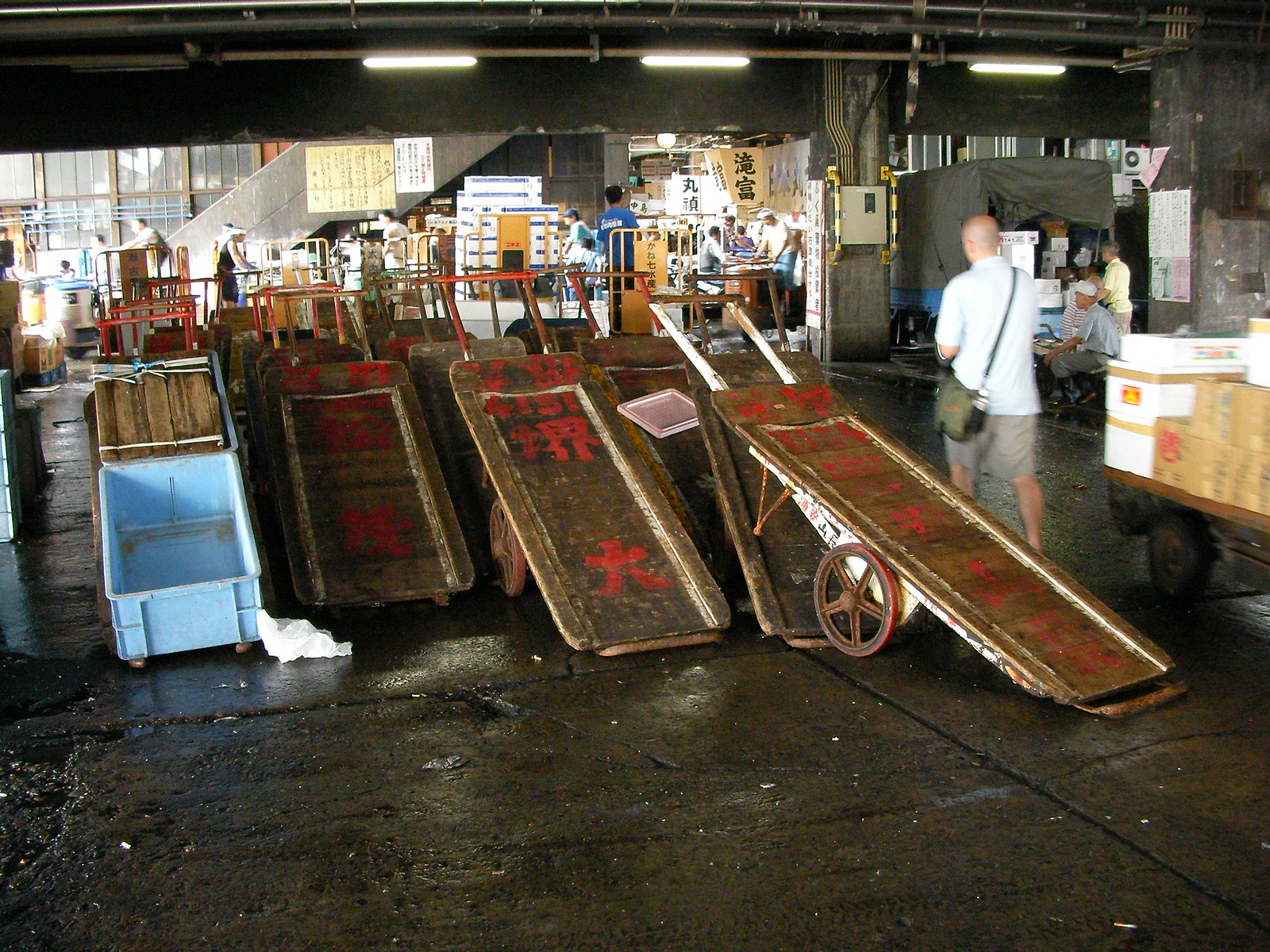The photograph captures an indoor scene within a bustling Asian factory, likely located in China. Centrally featured are several wooden flatbed carts, resembling wheelbarrows but with flat wooden tops and two large wheels each. Red Chinese characters cascade down the lengths of the carts. Approximately 10 to 12 carts are lined up in rows, creating a sense of organized chaos. A bald, white man wearing brown shorts, a white shirt, and a green crossbody bag walks past the carts. Around him, several factory workers are engaged in their tasks, pushing other loaded metal carts and moving boxes back and forth. The factory is brightly lit by fluorescent lights, casting reflections on the damp, dirty concrete floor which contrasts with the busy atmosphere. In the background, out-of-focus workers are seen amidst a maze of industrial activity, contributing to the vibrant industrious environment.